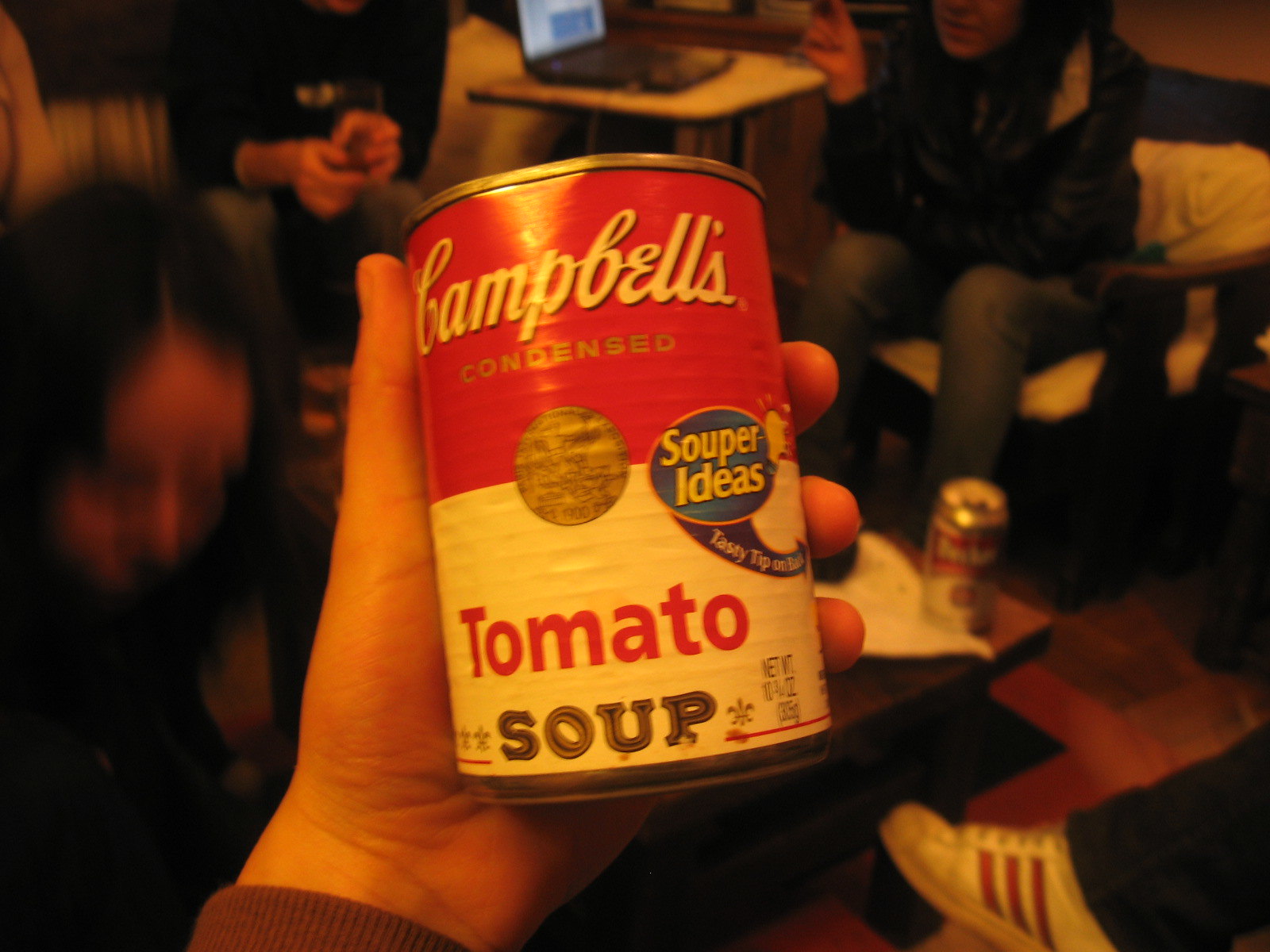A young man’s left hand, with fair skin, is prominently featured in the foreground, grasping a can of Campbell's tomato soup. He is dressed in a ribbed, wine-colored long sleeve shirt, with the cuff just visible at his wrist. The soup can appears slightly dirty and worn. In the background, a small group of people is gathered around a coffee table. To the left, a blurry woman with dark hair and fair skin gazes downward. Behind her, another individual with fair skin is gesturing animatedly; he is dressed in blue jeans and a black long sleeve shirt. To the right, an individual sits in a sturdy dark brown wooden chair with a cream-colored cushion, clad in blue jeans and a dark long sleeve shirt. In the immediate background behind the soup can, someone is seated with their legs crossed, visible from the shins down, wearing dark navy blue jeans and white tennis shoes with red stripes.